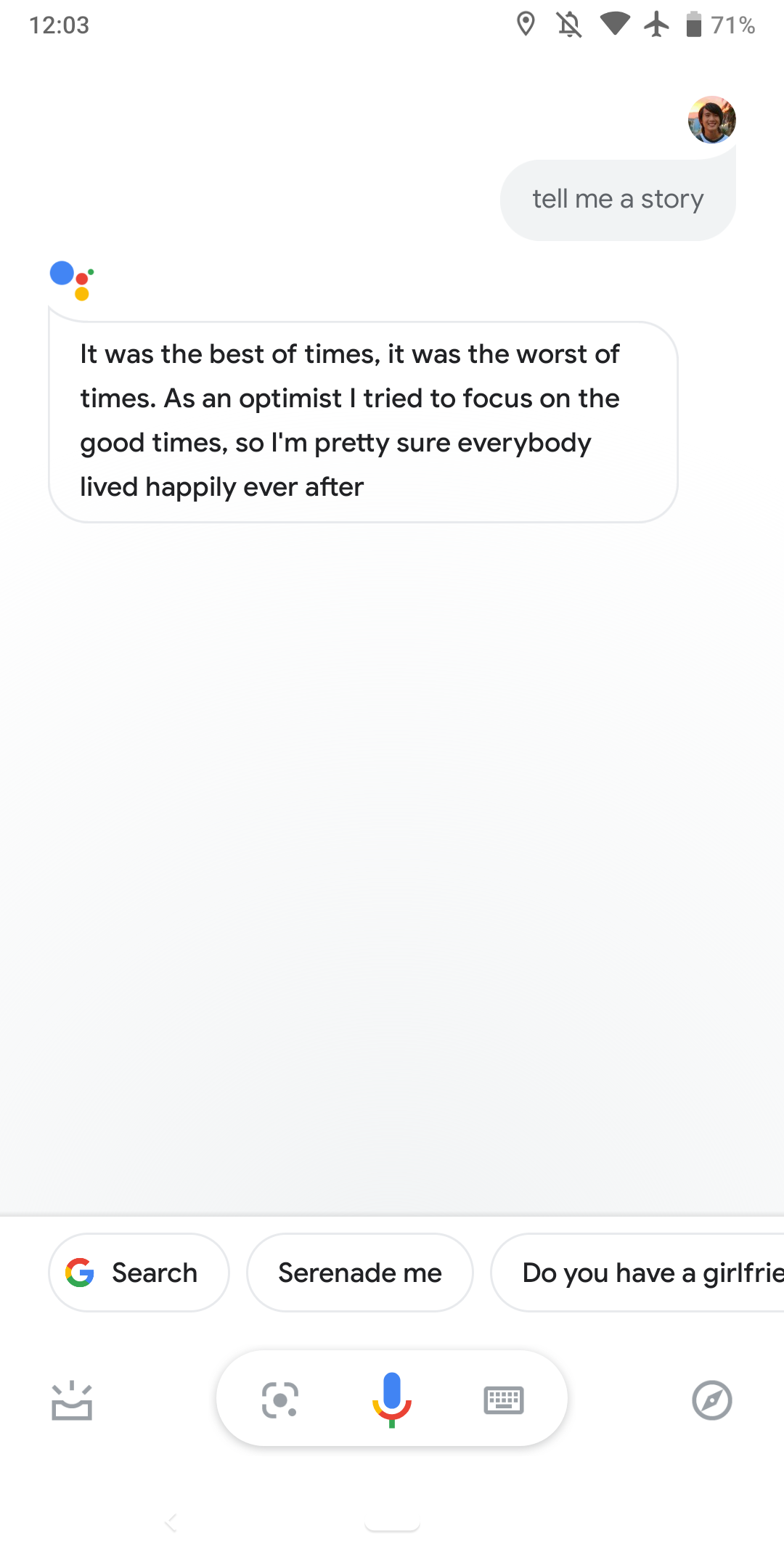Screenshot of a Mobile Device Using Google Assistant

The image is a detailed screenshot from a smartphone displaying an interaction with Google Assistant. At the top of the screen, the time is shown as 12:03 on a white background. Various status icons are visible, including a map pin, a bell icon with a slash indicating alarms are off, Wi-Fi signal strength, airplane mode activated, and a battery level at 71%. 

A user's profile icon is also present, depicting a person with short hair parted to the side, but the gender is indistinguishable. In the center of the screen, a Google Assistant query is shown with the text "Tell me a story." 

The recognizable Google Assistant logo, consisting of four colored circles in a pattern—blue (largest), red, yellow, and green (smallest)—is aligned to the left of the Assistant's response. The text narrated by Google Assistant reads, "It was the best of times, it was the worst of times. As an optimist, I tried to focus on the good times. So, I'm pretty sure everybody lived happily ever after."

At the bottom, Google Assistant provides three interactive options: "Search," "Serenade me," and a partially visible option cutting off with "Do you have a girlfriend?" Additional icons below these options include inbox, Google Image Search, voice input, a keyboard, and a compass for navigation.

The majority of the interface is presented against a simple white background, keeping the user interface clean and uncluttered.